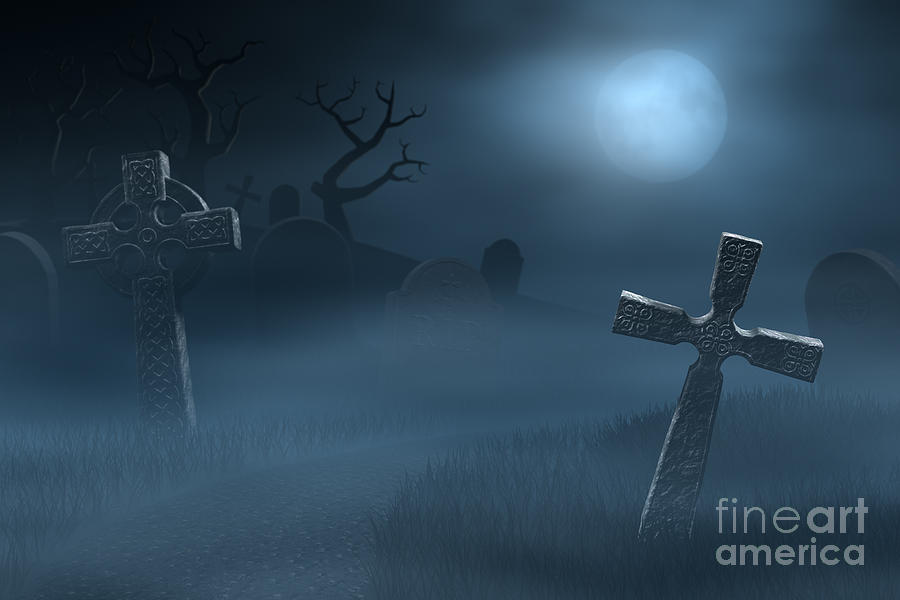This hauntingly atmospheric color illustration depicts a foggy graveyard at night, rendered primarily in tones of black, gray, and white. Dominating the scene are two elaborate metal crosses in the foreground; one leans to the right while the other tilts to the left, each adorned with intricate Celtic carvings. Scattered throughout the overgrown grass are various tombstones, with a few inscribed with "Rest in Peace" or "RIP." In the background, a hill rises with two gnarled, bare trees stretching towards the sky, their limbs reaching over the gravestones below. The full moon, partially obscured by a hazy, almost foggy cloud, casts a soft light across the eerie landscape. A barely defined dirt path meanders through the graveyard, adding to the sense of abandonment. In the bottom right corner, in all lowercase text, is the watermark "fine art america." The image exudes an otherworldly stillness, devoid of any people or animals.